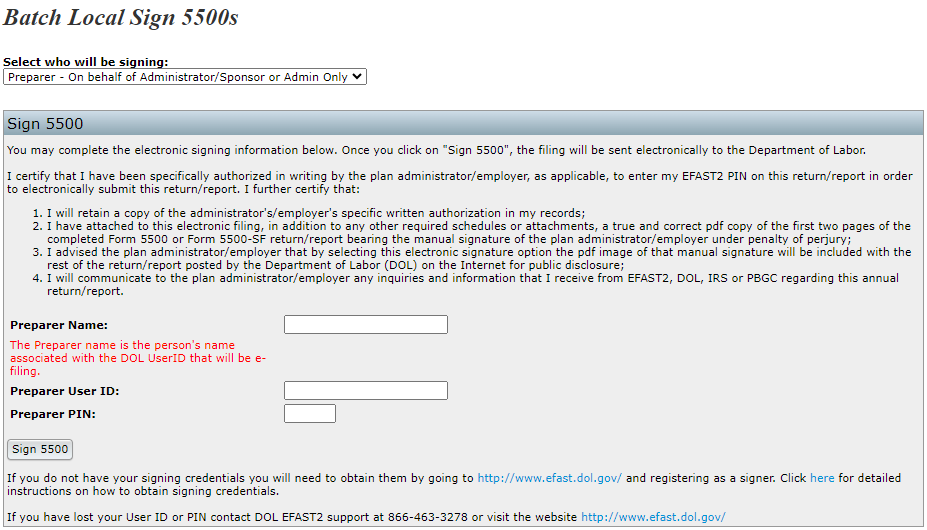The image depicts a digital interface for signing Form 5500 electronically. At the top, there's a section labeled "Batch Local Sign 5500s" and a prompt that reads "Select who will be signing." This prompt includes a dropdown menu with options: "Prepare on behalf of Administrator/Sponsor" or "Admin Only."

Below this, a gray box contains detailed signing instructions. The box header reads "Sign 5500." The instructions state that you may complete the electronic signing information below, and once you click "Sign 5500," the information will be sent electronically to the Department of Labor.

The text within the box provides a certification statement. It certifies that the individual has been authorized in writing by the plan administrator/employer to use their EFAST2 PIN to submit the return/report electronically. The signer must:
1. Retain a copy of the written authorization.
2. Attach a true PDF copy of the first two pages of the signed Form 5500 or Form 5500-SF, alongside any other required documents.
3. Inform the plan administrator/employer that by selecting electronic signature, the manual signature PDF will be publicly disclosed by the Department of Labor.
4. Communicate any inquiries from EFAST2, DOL, IRS, or PGC to the plan administrator/employer.

Below the instructions, there's a section to enter the "Preparer Name" in red, which will be associated with the DOL user ID for e-filing. Next to this, there is an empty box where the user must enter the "Preparer User ID," and another box to the right for the "Preparer PIN."

At the bottom, there's a "Sign 5500" button. Additional guidance is provided if the user does not have their signing credentials, directing them to visit http://www.efast.dol.gov for registration or detailed instructions. For those who have lost their User ID or PIN, the document advises contacting DOL EFAST2 support at 866-463-3278 or visiting the aforementioned website.